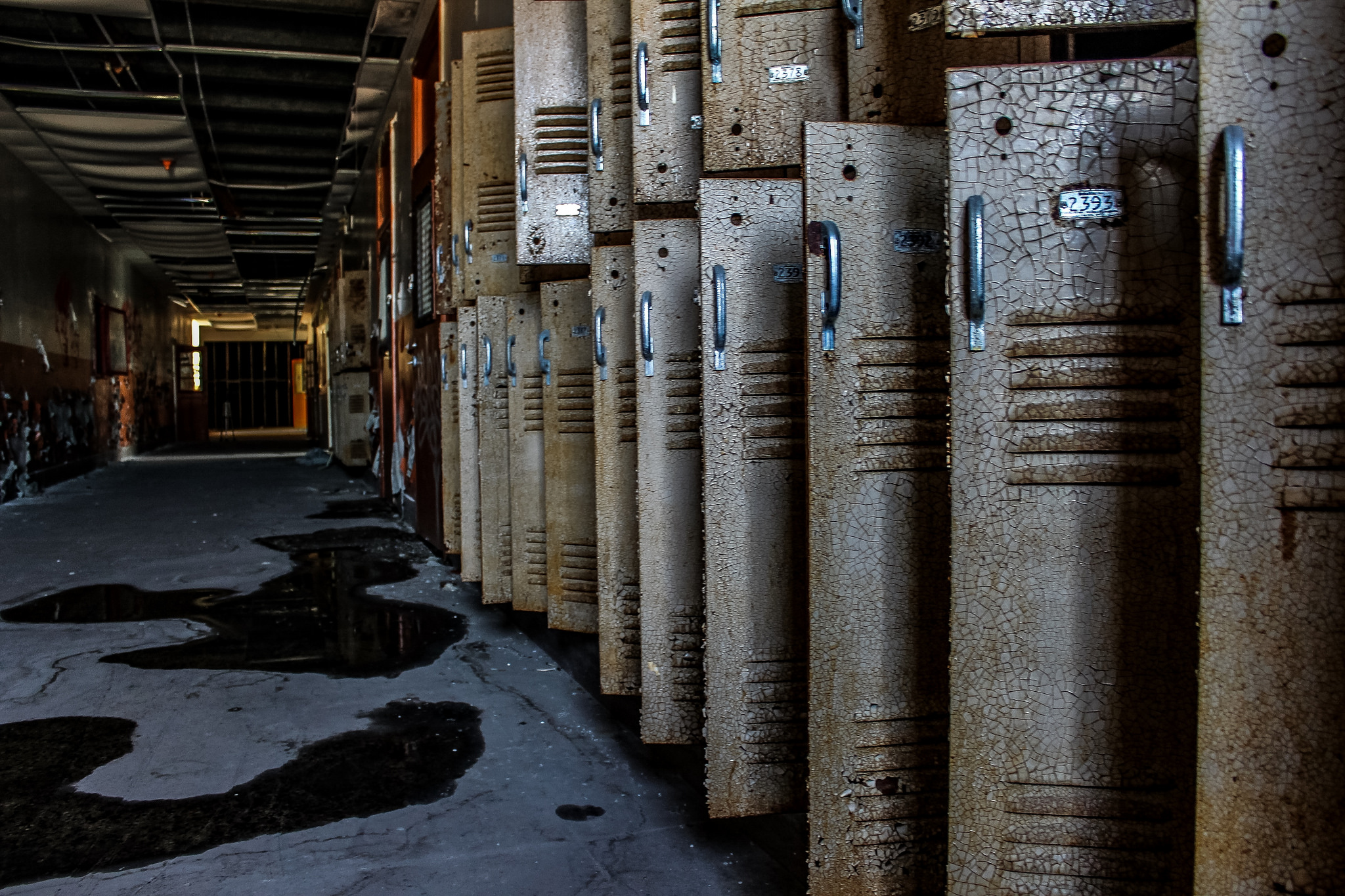This image depicts a desolate, abandoned school hallway, shrouded in decay and neglect. The scene is dominated by two rows of rusting, tan-colored lockers on the right wall, all of which have their doors eerily ajar. Each locker features cracked and flaking paint, reminiscent of a lightning pattern, with silver handles located at the top left corner and two vent sections. Notably, one locker bears the number 2393. The gray cement floor is stained with dark puddles, hinting at water damage, while debris is scattered throughout the hallway. The ceiling above is in disrepair, missing numerous tiles and exposing the steel framework. At the far end of the hallway, a faint light filters through an open red door, adding to the tunnel-like effect of the dim corridor. This haunting image, accentuated by the interplay of natural light and shadows, evokes a sense of eerie abandonment, as if straight out of a horror movie.